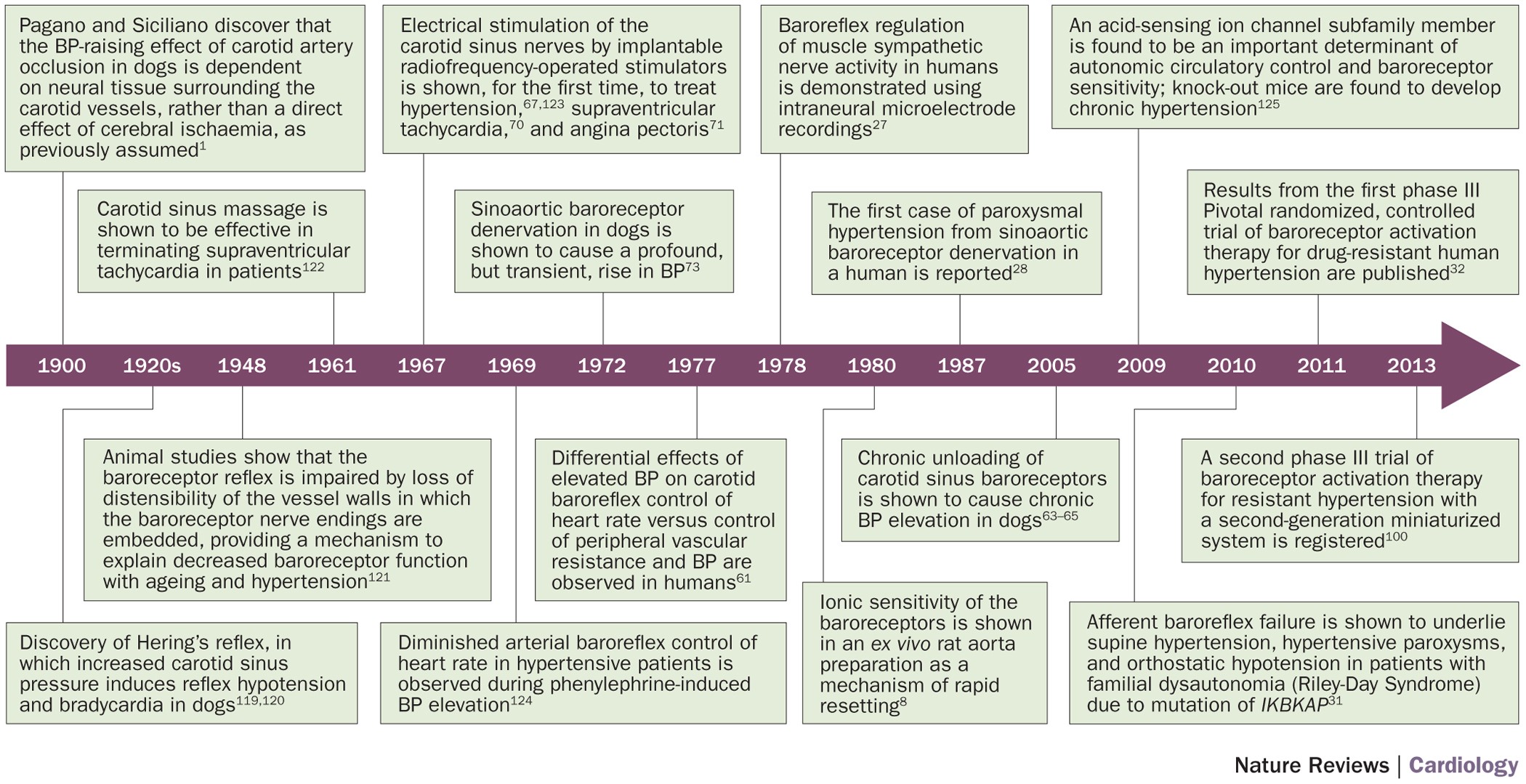This is a detailed scientific timeline depicted in a graphic format, focusing on advancements in cardiology from 1900 to 2013, as reviewed by Nature Reviews Cardiology. The central element is a long, narrow maroon arrow pointing to the right, with significant years marked in white text including 1900, 1920s, 1948, 1961, 1967, 1969, 1972, 1977, 1978, 1980, 1987, 2005, 2009, 2010, 2011, and 2013. Branching off this arrow are numerous lines connecting to greenish text boxes, each box filled with detailed information about historical events and discoveries in cardiology for the corresponding years. The diagram is comprehensive, featuring a total of sixteen text boxes aligned in rows both above and below the main arrow, each elaborating on key scientific findings and medical advancements, such as the chronic unloading of carotid sinus baroreceptors causing chronic blood pressure elevation in dogs. The detailed and dense nature of the text suggests a strong focus on the biological and medical intricacies related to cardiology.